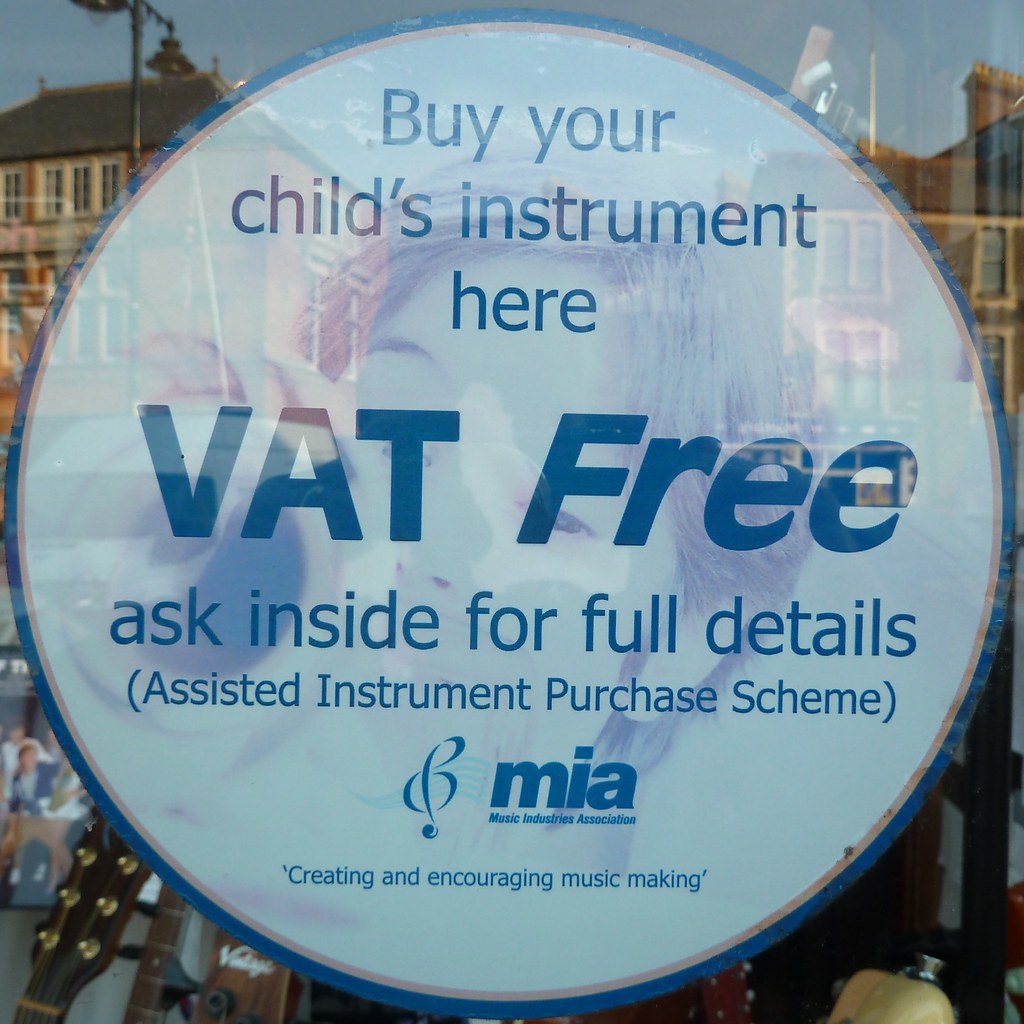In the image, we see a detailed advertisement displayed in the window of a music store. The focal point is a large, round sign with a white background and a blue border encircling it. Prominently printed in blue text, the sign reads, "Buy your child's instrument here." Below this, in bold blue letters, it declares, "VAT free," followed by the instruction, "Ask inside for full details." Parenthetically, the words "assisted instrument purchase scheme" are included. 

Additionally, the sign features a logo of a treble clef next to the acronym "MIA," denoting the Music Industries Association, accompanied by the slogan, "Creating and encouraging music making." The reflection in the glass reveals a cityscape with large, older colonial-style buildings, alongside a glimpse of the store's interior, where you can spot the fretboard and tuning area of a guitar. A subtle backdrop image of a child playing a trumpet adds a nostalgic touch to the advertisement.